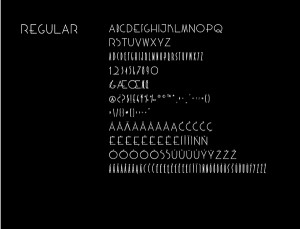The image features a black square background with very thin, light gray text and lines. In the upper left corner, in a fancy, capitalized font, the word "REGULAR" is displayed. 

Centered at the top, the entire alphabet is showcased in this elegant, calligraphic font. Just below the alphabet, there's a series of straight horizontal and vertical lines. Further down, a set of thin numerals appears.

Beneath the numbers, a few individual characters such as '6', 'A', and 'C' can be seen, followed by various symbols including the '@' symbol, an asterisk (*), and commas.

In the following row, the letter 'A' is repeated numerous times, while the next row features the letter 'C' repeated about five times. The next subsequent row contains multiple letters 'E'. Moving down, you can see a series of letters 'O', 'U', and 'Y' repeated twice, with the letter 'Z' repeated three times. Finally, the bottom row consists exclusively of horizontal lines.